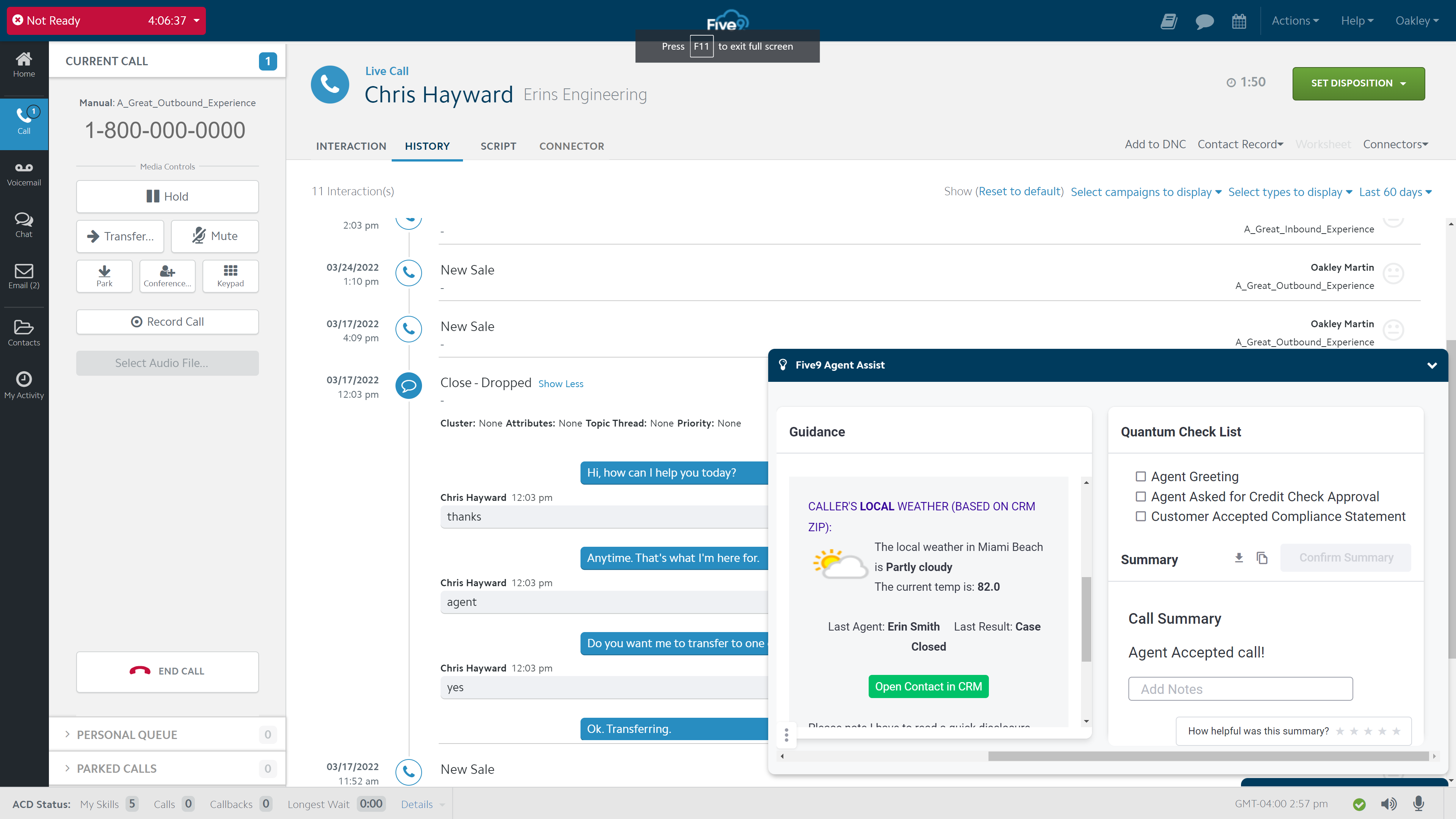This is a screenshot of a website for "Five Five Nine." On the left-hand side, there is a narrow vertical sidebar with seven icons. At the top of this sidebar is the Home icon, followed by the Core icon. Below these, the options include Chat and Contacts. 

To the right, the main screen displays the Core section, showing a phone number 1-800-000-0000. Directly beneath the number, media control options are visible, allowing the user to hold, transfer, mute, and record the call. 

The main interface indicates an ongoing live call, with a duration of 1 minute and 50 seconds elapsed. The call is with Chris Heywood from Errands Engineering. The currently highlighted tab is the History tab, providing access to past interactions.